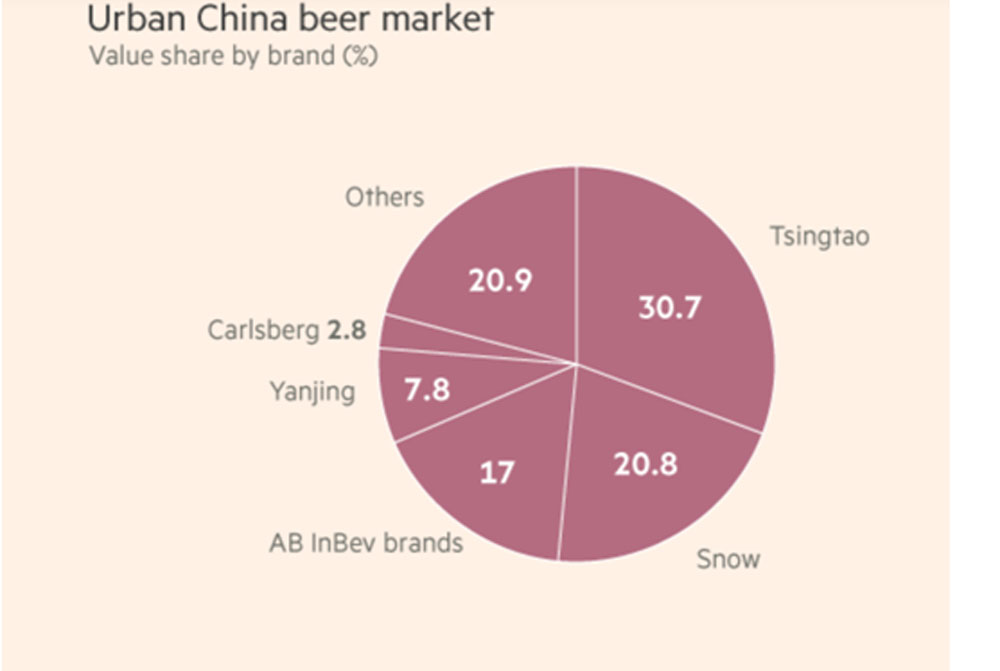The image features a detailed pie chart on a pale yellow background, representing market share data for various beer companies in Urban China. At the top left, in black text, the chart is titled "Urban China Beer Market," followed by a subtitle, "Value Share by Brand (%)". The pie chart itself, colored in shades of purplish-red with sections labeled in white, segments market share distribution among several beer brands. Tsingtao leads with 30.7%, followed by Snow with 20.8%, while "Others" comprise 20.9%. Additional segments include AB InBev Brands at 17%, Yanjing at 7.8%, and Carlsberg with the smallest share of 2.8%.